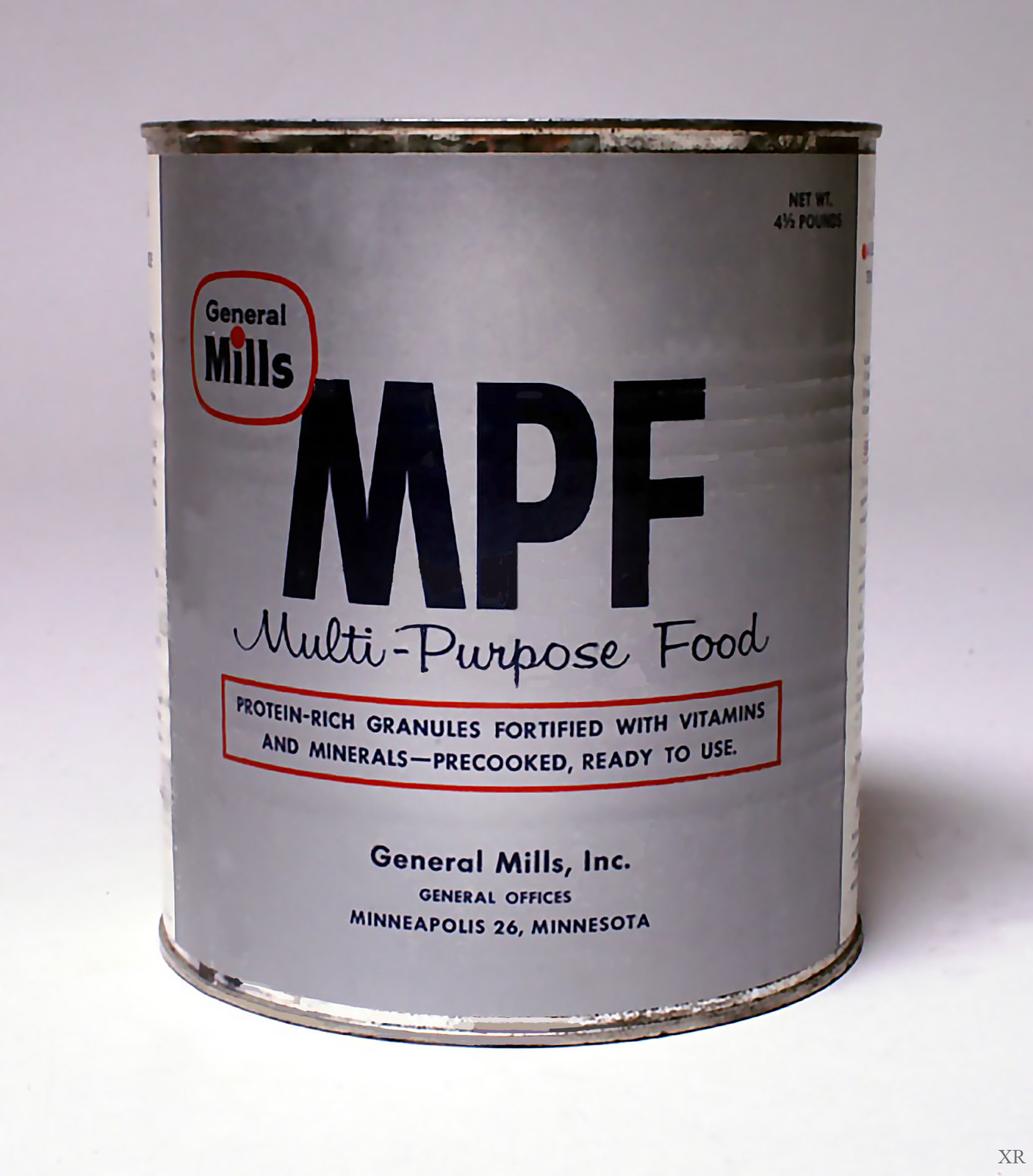This color photograph showcases an old General Mills multi-purpose food (MPF) can. The can is set against a plain white background, emphasizing its features. It is primarily light gray with silver metal at the top and bottom, both showing signs of rust and wear. The label is detailed, with a red circled logo of "General Mills" in the upper left corner. To the right of the logo, prominent black letters spell out "MPF." Below this, in cursive, it states "multi-purpose food." Further down, a red-outlined rectangle contains the text: "Protein-rich granules fortified with vitamins and minerals, pre-cooked, ready to use." At the bottom of the label, it reads: "General Mills Incorporated, General Offices, Minneapolis, 26th Minnesota." The can also features ribbed bands designed for an easier grip.